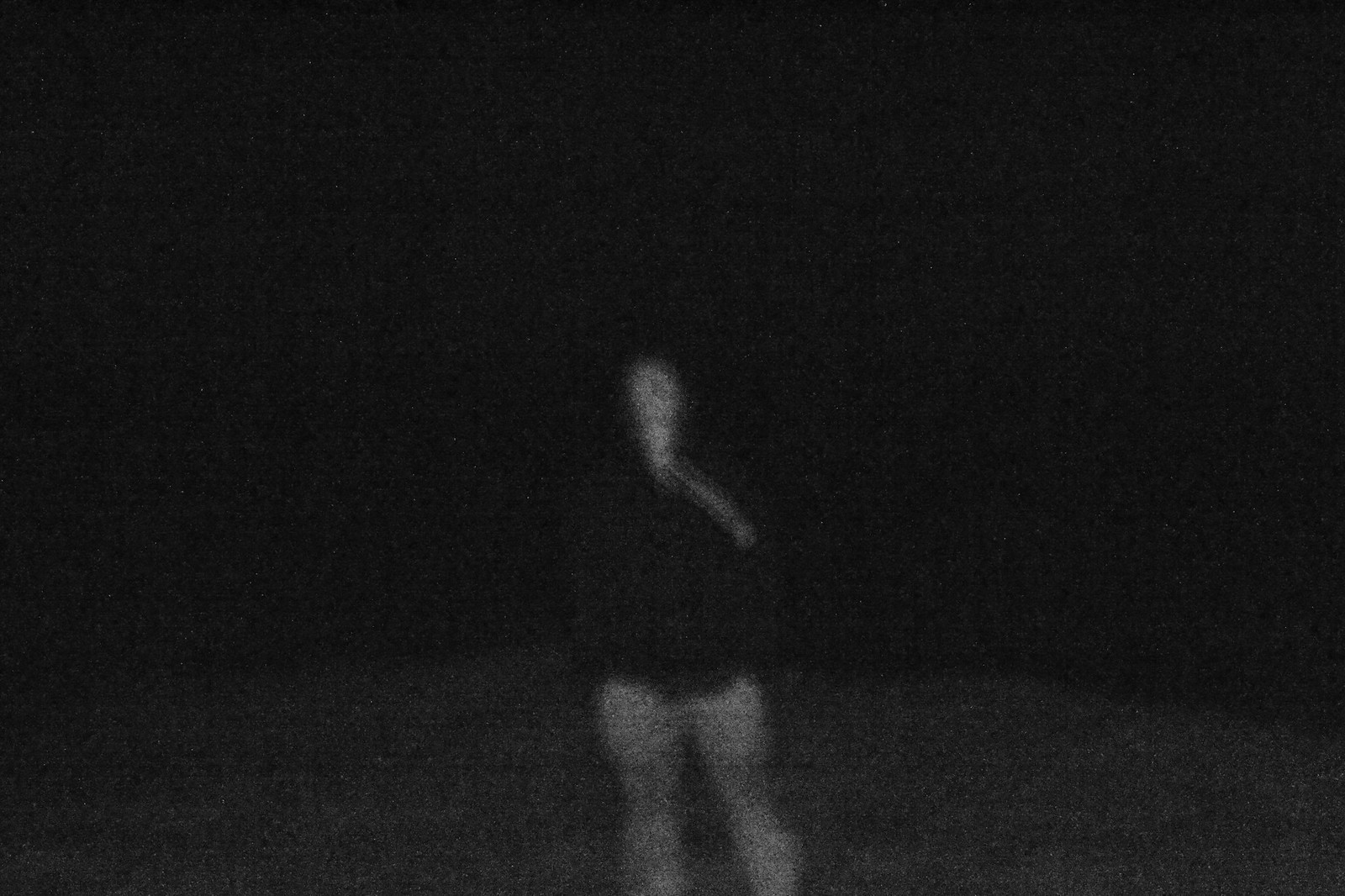This nighttime outdoor photograph captures a solitary figure against a predominantly black backdrop. Positioned centrally in the lower half of the horizontal frame, the person is nearly camouflaged due to their dark attire. The dimly-lit background is filled with gradients of dark gray, creating a foreboding atmosphere. The figure's clothing suggests they are wearing shorts, revealing their thighs, knees, and calves, although their feet are cropped out of the composition. The individual's face and neck are rendered in a spectral light gray, devoid of discernible details and possibly angled upwards as though gazing at the stars. A subtle, narrow line of darker gray extends from the neck to the lower right, implying the person's left hand is raised slightly above shoulder level. The overall image is characterized by its stark contrasts and eerie, minimalistic aesthetic.